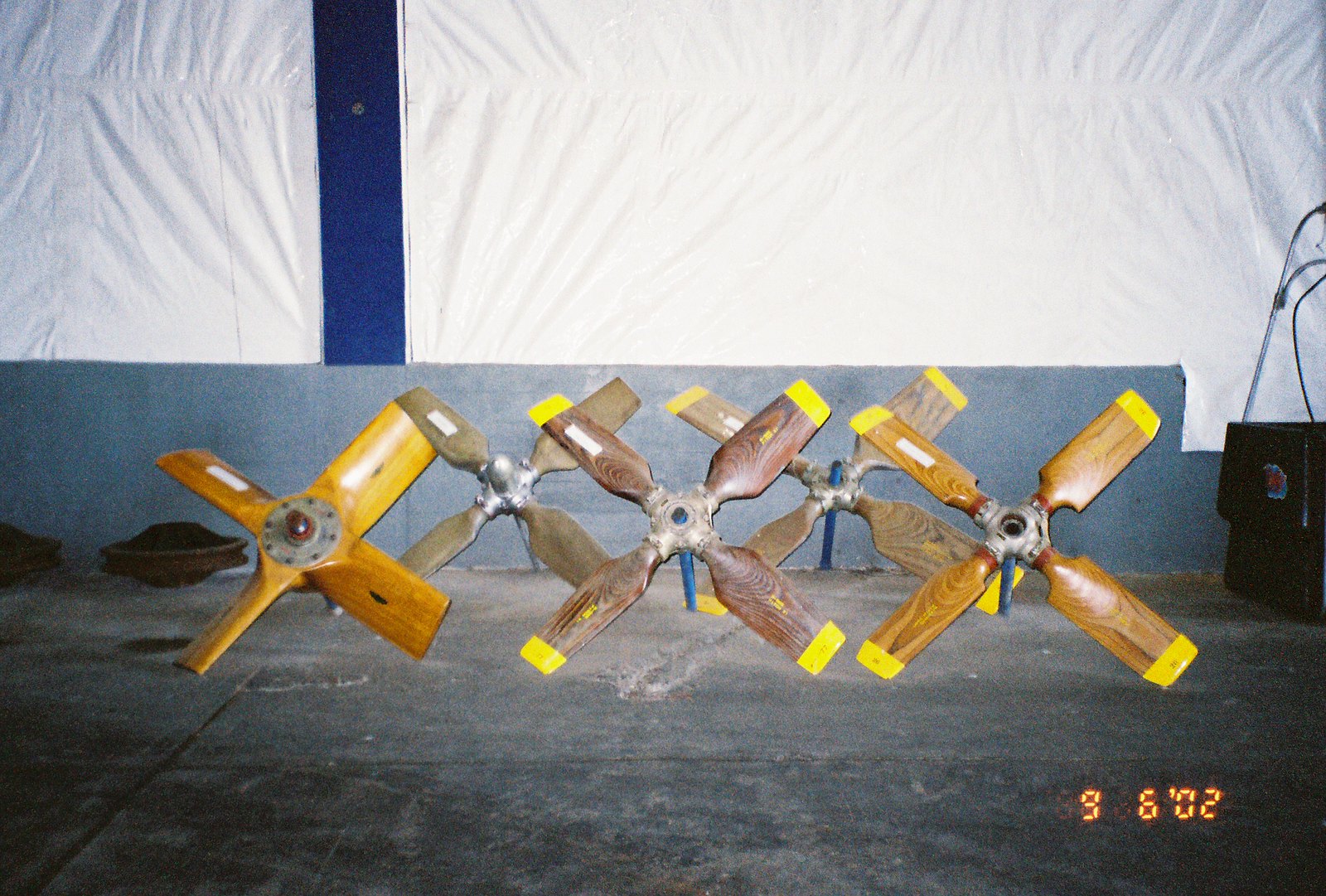In this detailed image, there are five wooden airplane propellers arrayed against a large blue wall adorned with a white banner, which features a single blue streak slightly off-center to the left. The propellers, each with yellow-tipped blades, exhibit various shades of wood from light to dark, highlighting their distinct grain patterns. They are uniformly equipped with metal circular connectors at their centers and are supported by a blue shaft positioned behind them. The propellers rest on a concrete hangar floor, propped up on their blades while the blue shaft ensures they are angled upward. In the background, some rusted metal saucers lie to the back left, and additional equipment is visible to the right. The image also includes some numbers, 9-6-0-2, in the bottom corner.